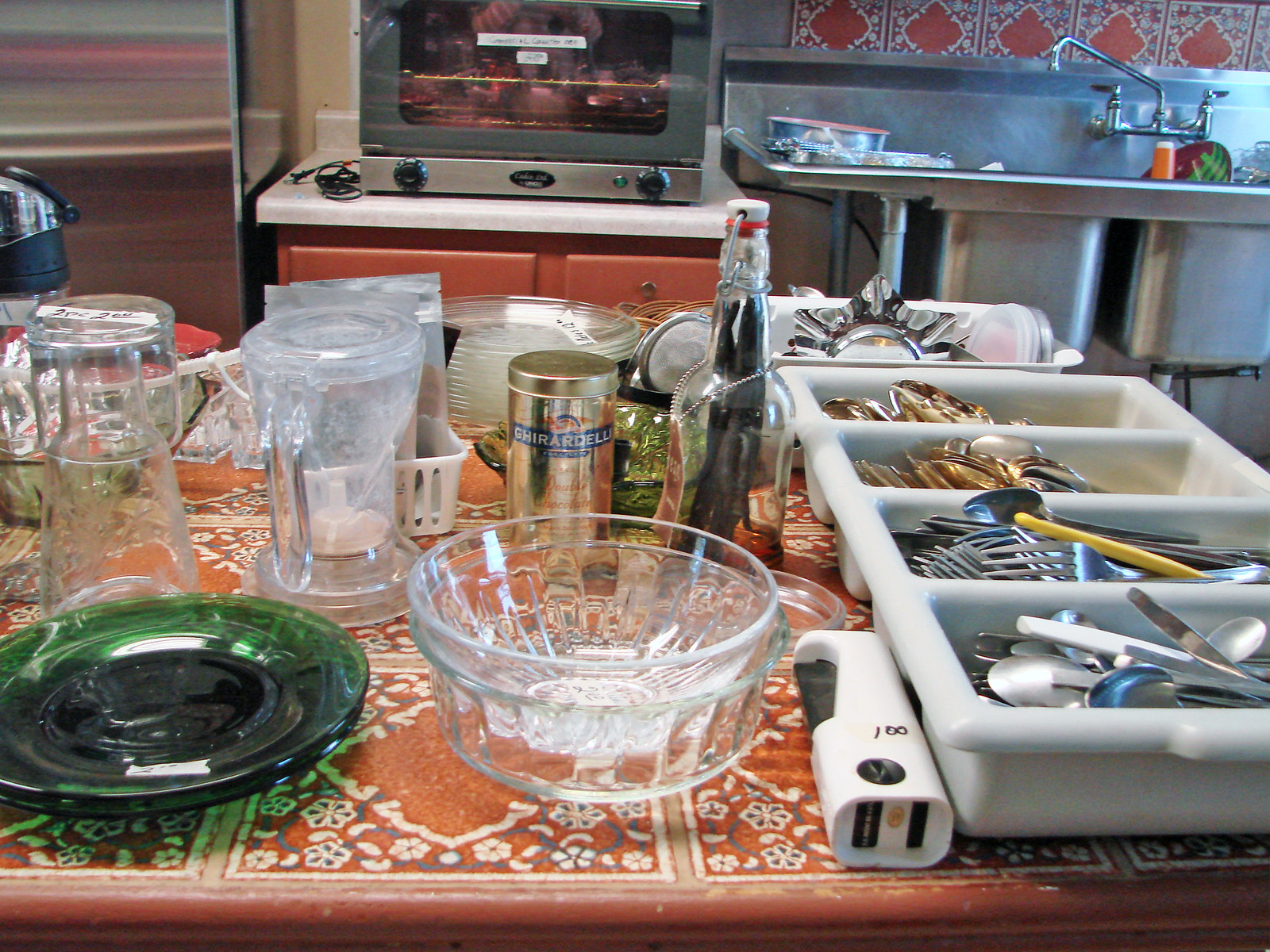The image depicts a bustling kitchen that appears to be in the midst of either preparation or cleanup after cooking or baking a substantial meal. The setting is reminiscent of a professional space due to its industrial elements, but possesses a homey vibe that hints it might belong to a residential setting.

In the background, an industrial-style, stainless-steel double-basin sink occupies the very far wall. Although such a sink is commonly found in restaurant kitchens, this one is surrounded by elements that suggest a home setting. The wall behind the sink is adorned with a dated, yet captivating, Middle Eastern pattern. The intricate design features deep rust-red hues with paisley-like details, evoking a 1970s aesthetic.

To the left of the sink, an unplugged industrial-style toaster oven sits with its cord neatly coiled beside it. Central to the image is a heavily laden table, covered in the same Middle Eastern pattern that decorates the wall, possibly hinting at a thematic design or a coordinated interior decor.

The table, chaotic and crowded, is the focal point of the picture. To the right, there are several bins of silverware arranged in a straight line, starting with spoons closest to the viewer, followed by forks. Interestingly, after the silver utensils, there are bins containing gold-colored spoons, adding to the eclectic mix. 

Scattered across the table are a variety of items: a glass bowl adjacent to a green plate, a bottle of liqueur, and a package of Ghirardelli chocolate, suggesting either recent or upcoming culinary activities. Additionally, various sized plates, vases, and containers add to the clutter, creating a scene that mirrors the organized chaos typical of a kitchen in full holiday preparation mode.